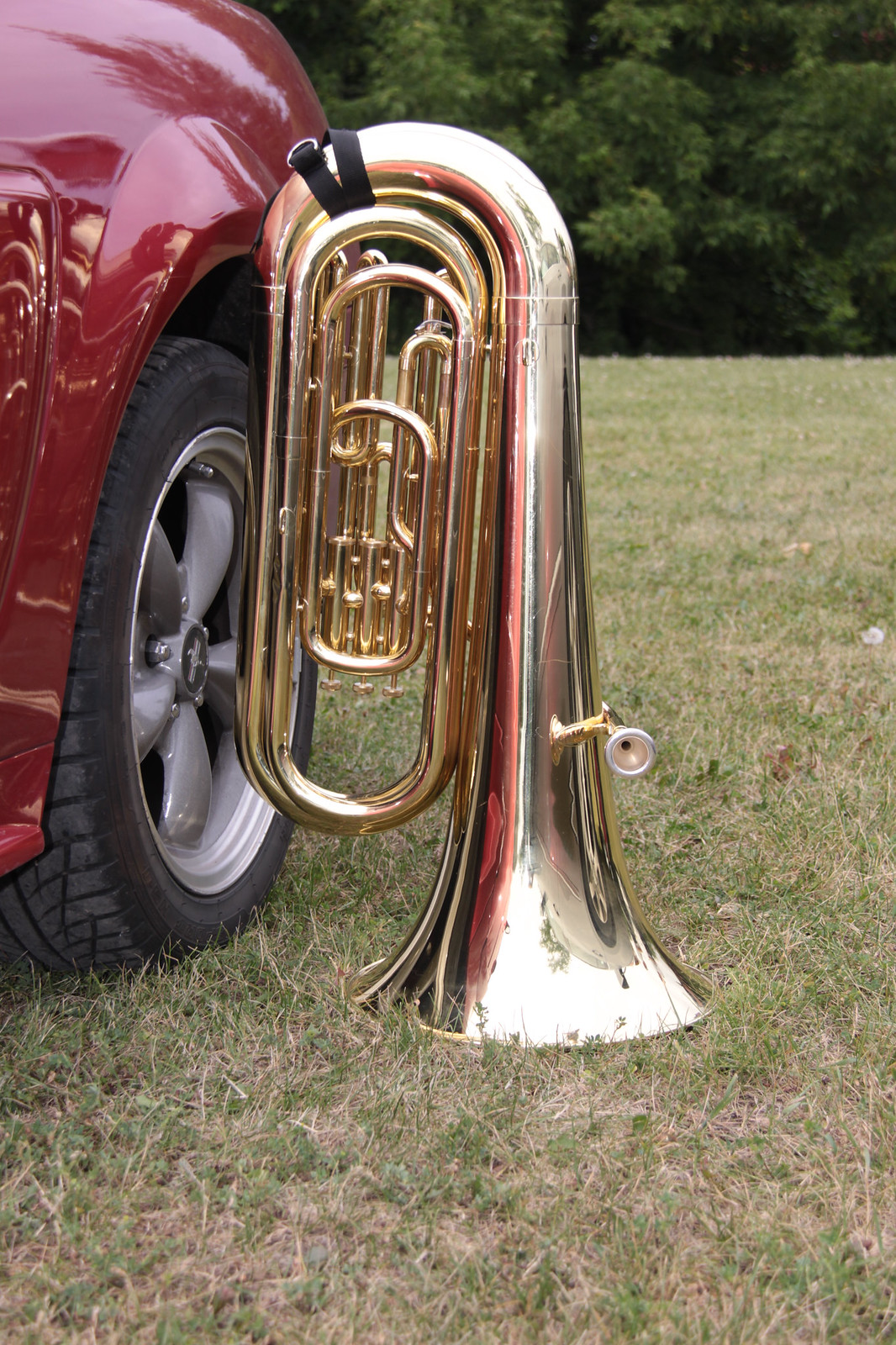A silver trombone with reddish trim and a brass-colored midsection is seen standing upright on browning grass next to the rear tire of a shiny, reddish-purple car. The curved bell of the trombone is inverted, and the silver mouthpiece is prominently attached. A black strap is located near the top left of the instrument. In the background, tall green trees frame the scene in an expansive and clear field.